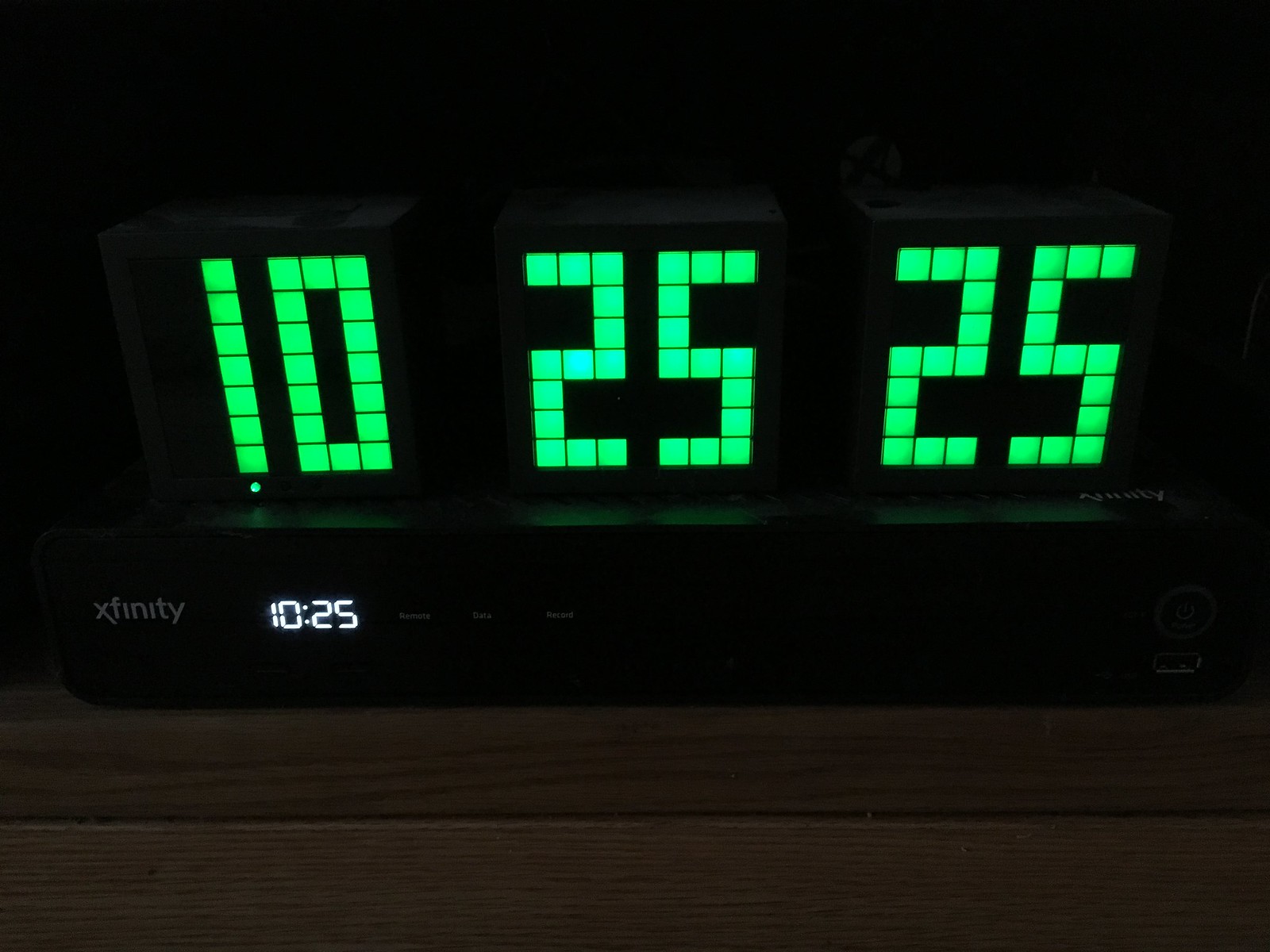The image features a jet black background with digital numbers prominently displayed in lime green, composed of individual square pixels. These numbers, aligned from left to right, are 10, 25, and 25, representing hours, minutes, and possibly seconds, respectively. Below these large green numbers, in smaller white pixels, the time reads 10:25. To the left of the white digits, the name "Xfinity" appears in small gray letters. A faint reflection can be seen underneath the large green digits, suggesting a sheen on the black surface below. Surrounding the bottom of the display is a framed or raised edge, and the entire device appears to be placed on a wood-colored surface, enhancing its sleek, modern aesthetic.